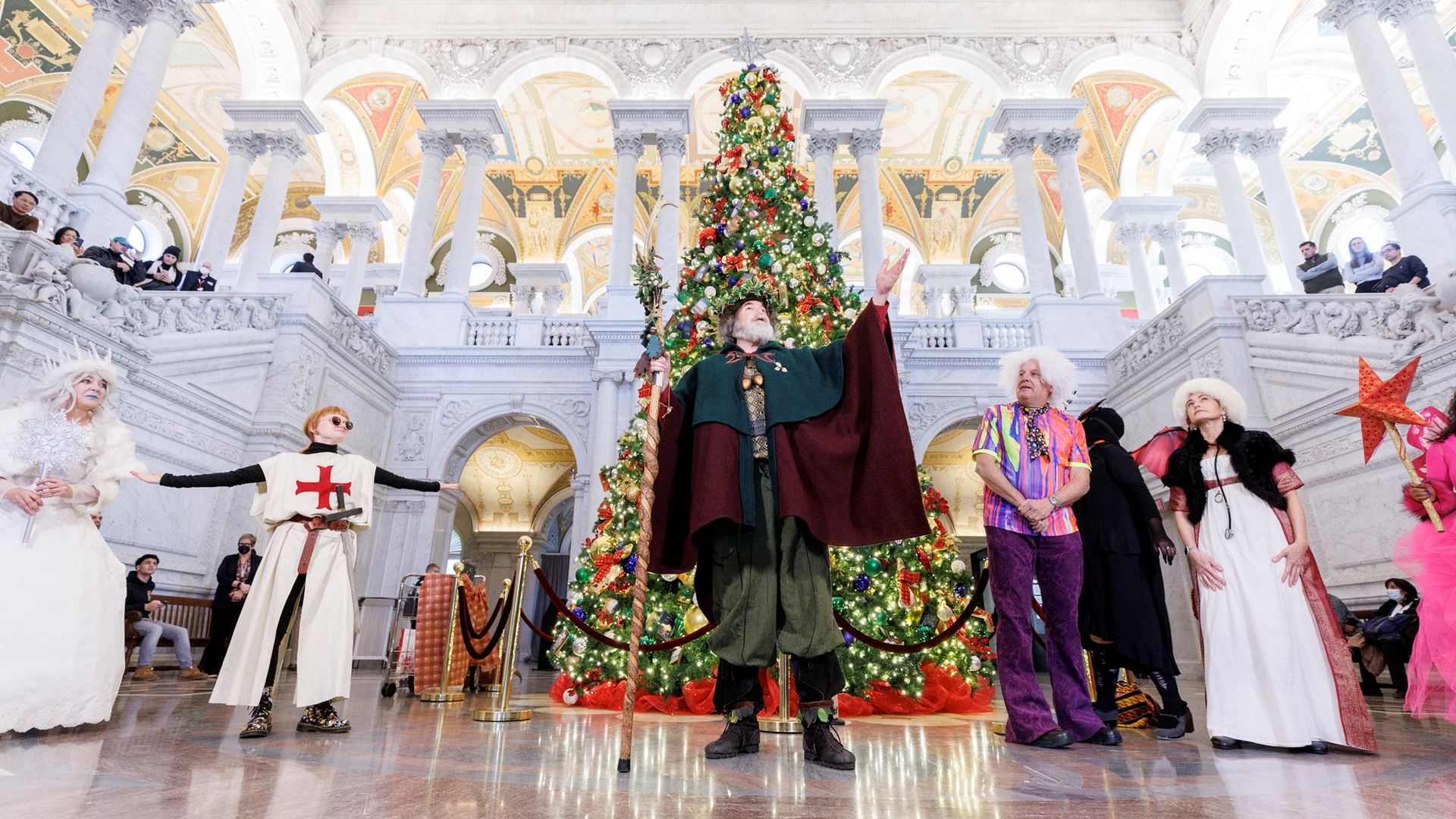In this ornate, palace-like setting resembling an elegant, historical chapel or a mall, a festive Christmas celebration unfolds. The scene is framed by gleaming, double-columned pillars and archways with intricate designs, creating a grandiose atmosphere. From the ground floor, with its shiny granite surface, we gaze upward to include multiple floors where onlookers gather at the stairwells and balconies, some appearing to be singing.

At the heart of the scene, a colossal, ornately decorated Christmas tree stretches almost to the ceiling, adorned with numerous decorations and encircled by a protective rope. In front of this majestic tree stands an elderly man of Caucasian descent, embodying an Old World Father Christmas. His attire includes a green and maroon cloak, baggy green slacks, and black boots. He sports a crown of green holly leaves atop his white beard and holds a wooden walking stick in his right hand, while his left hand is extended upward and outward as he gazes before him.

To the left of Father Christmas is a figure in crusader attire, wearing a white tunic with a red cross over a long-sleeved black turtleneck and black pants. Further left is a woman with white hair, styled to resemble a crown of snow or ice with icicles, donning a pure white dress and blue lipstick, and holding a wand shaped like a snowflake. To the right of Father Christmas stands another older man with fluffy white hair, wearing purple pants and a striking purple-striped shirt with hints of green and orange. Finally, to the far right, there's a lady in white with a fur coat, turned slightly away from the camera. The combined elements of this spectacularly detailed indoor scene capture the essence of a lavish holiday celebration.